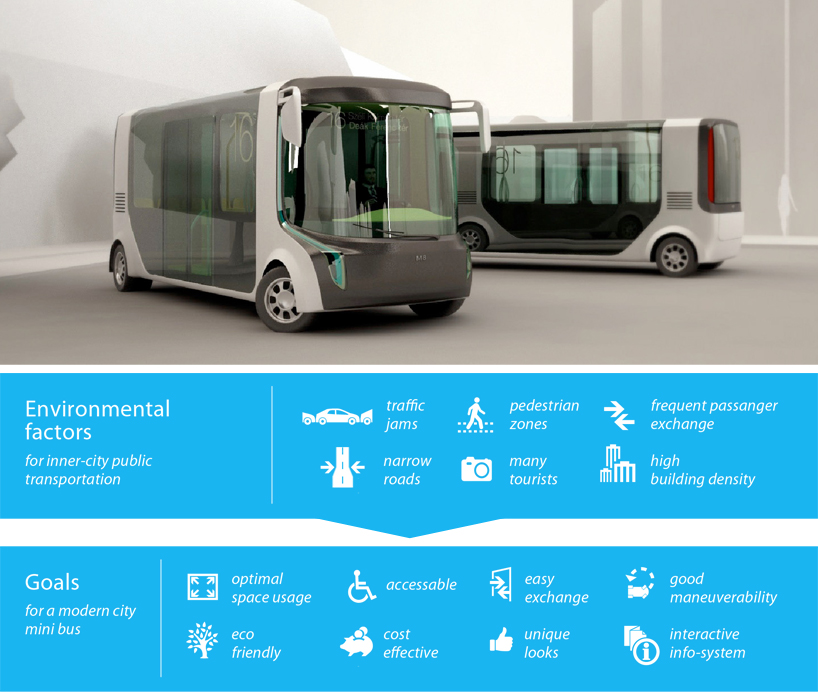The poster features two futuristic electric minibuses, designed for inner-city public transportation. These vehicles, likely intended for passenger transport, resemble mini buses with elongated and wider bodies compared to your average minivan, accommodating approximately 10 to 12 passengers. They are characterized by their small wheels, low-profile bodies, and largely glass sides. Each bus has minimalistic bumpers and large white side mirrors. 

The foreground bus, marked with the number 16, has its steering wheels turned to the left. The other bus in the background faces the opposite direction, suggesting it is parked. These details are set against a gray concrete surface with a backdrop consisting of gray and white walls, creating a modern and sleek aesthetic.

Below this image, a section labeled "Environmental Factors" is displayed on a blue background with white text. It lists critical considerations for inner-city public transportation such as traffic jams, narrow roads, pedestrian zones, high building density, numerous tourists, and frequent passenger exchanges.

Furthermore, the goals detailed for these modern electric minibuses include optimal space usage, eco-friendliness, wheelchair accessibility, cost effectiveness, ease of exchange, unique appearance, good maneuverability, and an interactive info system. This emphasis on advanced features and eco-friendly design portrays these electric minibuses as innovative solutions for future urban transport challenges.